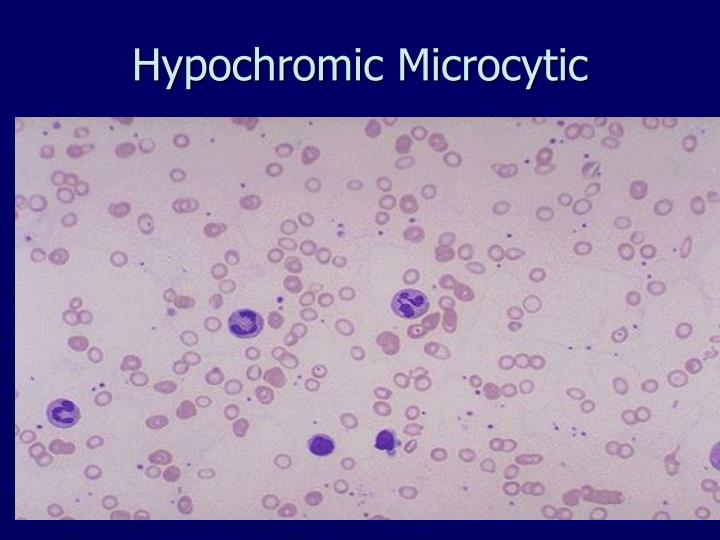The image features a blue and pinkish-purple background with the text "Hypochromic Microcytic" in all white letters at the top, capitalizing the 'H' and 'M'. Encased in a dark blue border, the main focus lies on numerous cell-like structures scattered across a light purple and blue-gradient backdrop. The majority of these cells are light purple circles with some darker dot purples interspersed. There are five notably larger cells with a darker purple hue, each having even darker purple blotches within them; these prominent structures are mainly situated towards the left. The composition and distribution of these cell-like items suggest a scientific or microscopic setting, emphasized by the meticulous detailing and organized randomness within the image.